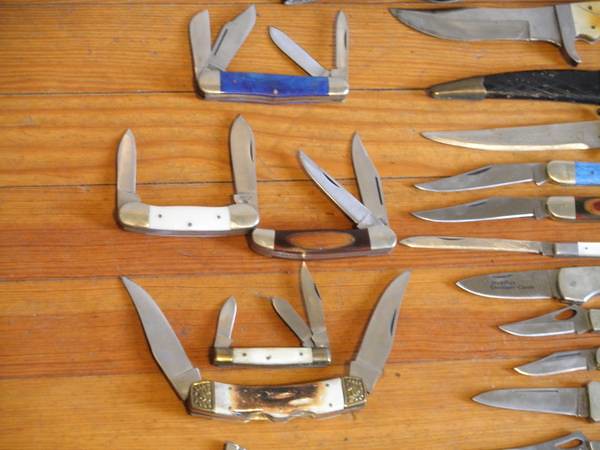This detailed photograph captures a top-down view of a light brown wooden table adorned with an array of pocket knives and multi-tools. The collection includes knives of various designs, sizes, and colors, neatly laid out horizontally across the table. 

At the center, there are five distinctive folding knives, with one at the top featuring a blue handle and four blades extended at varying angles, illustrating their multifunctionality. Below this blue knife, there are two more knives placed side by side horizontally: a white-handled knife with blades extended from both ends, and a brown-handled one with two blades deployed on the right. Further down, there is a smaller folding knife with one blade extended to the left and two more to the right. At the very bottom lies an ebony-handled knife with a brown middle, featuring two blades extended from both ends, resembling the shape of a helmet, akin to Loki's from mythology.

On the right side of the table, there is a cluster of approximately ten to eleven knives, their blades prominently jutting out from the right edge of the frame, displaying varying degrees of sharpness and sizes. Some of these knives have handles adorned with mother-of-pearl and brass trims, highlighting their craftsmanship. Each blade has a distinct groove at the top, enabling easy use.

The repeated emphasis on the variety and detailed placement of each knife suggests that these items might have been confiscated. The collective display on the timber slat table creates a visually striking representation of diverse pocket knife designs and functionalities.